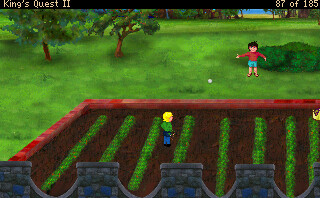This is a square-shaped image capturing gameplay from "King's Quest LL." In the top left corner, the game's title is displayed in clear white text. The top right corner shows the text "887 of 185," indicated in a vibrant yellow font. At the center of the image, a character with striking yellow hair is prominently featured, dressed in a green top and blue pants. The character stands in a field, which consists of brown dirt and verdant green plant lines crisscrossing the terrain. The scene suggests a natural environment brimming with foliage and a cultivated landscape.